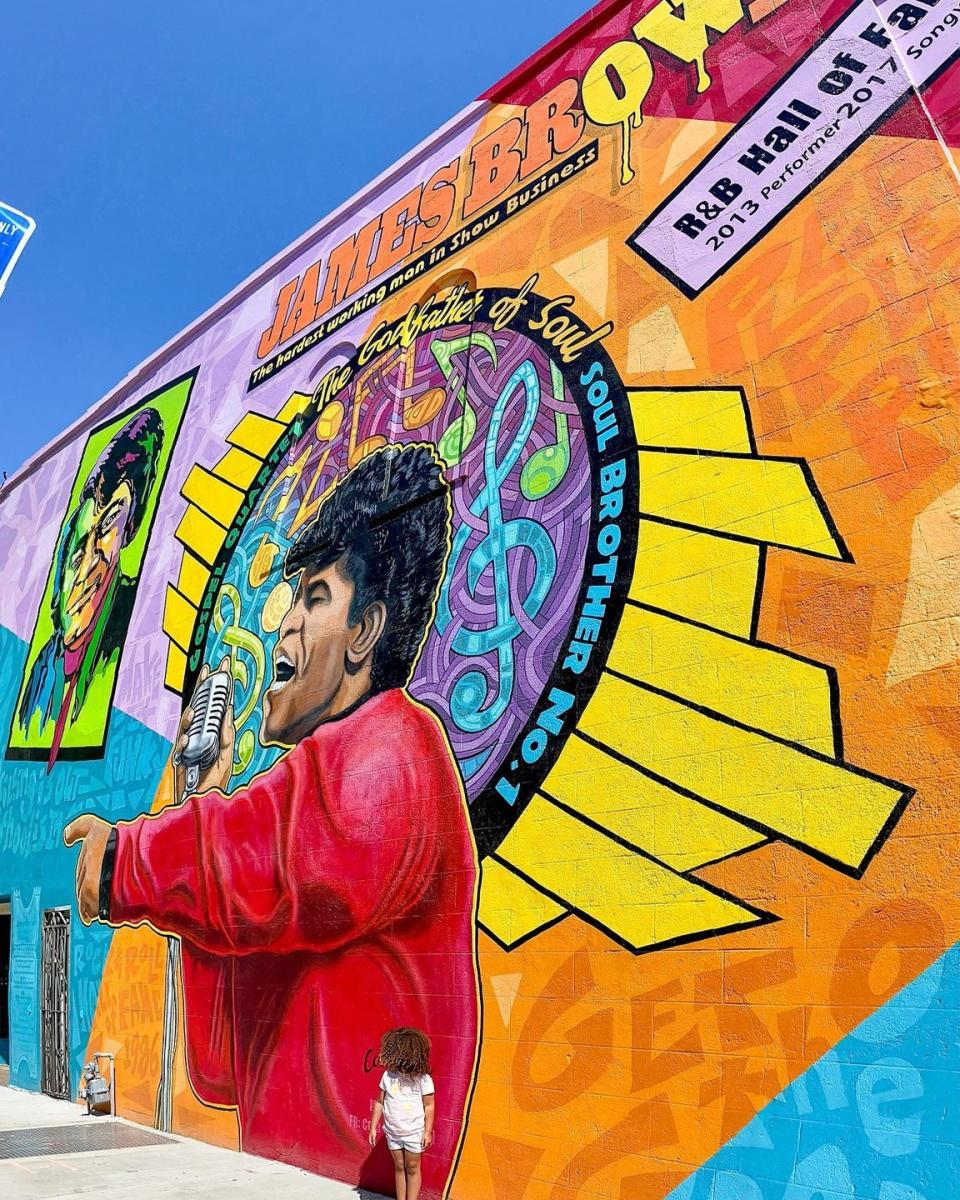In this photograph, we see a vibrant outdoor mural painted on the side of a four-story cinder block wall. The foreground features a small child with big, curly hair partially obscuring her face. She stands on a gray tiled sidewalk, dressed in a white t-shirt and white shorts.

Dominating the mural is an energetic depiction of James Brown, famously known as the "Godfather of Soul" and "The Hardest Working Man in Show Business." He is captured mid-performance, singing into a microphone, wearing a striking red jacket. Surrounding him is a black ring adorned with colorful musical notes and lines in hues of green, yellow, orange, blue, purple, and pink.

Above the mural, at the very top of the wall, bold letters spell out "James Brown." Additional text within the mural proclaims his titles and accolades, including “Soul Brothers Number One,” “R&B Hall of Fame 2013 (Performer),” and “2017 (Song).” The backdrop of the mural is equally captivating, with large, blocky shapes in colors like orange, pink, red, purple, and blue, creating a dynamic and lively scene. To the upper left of the mural, the clear blue sky peeks into the frame, adding to the sense of scale and openness in the image.